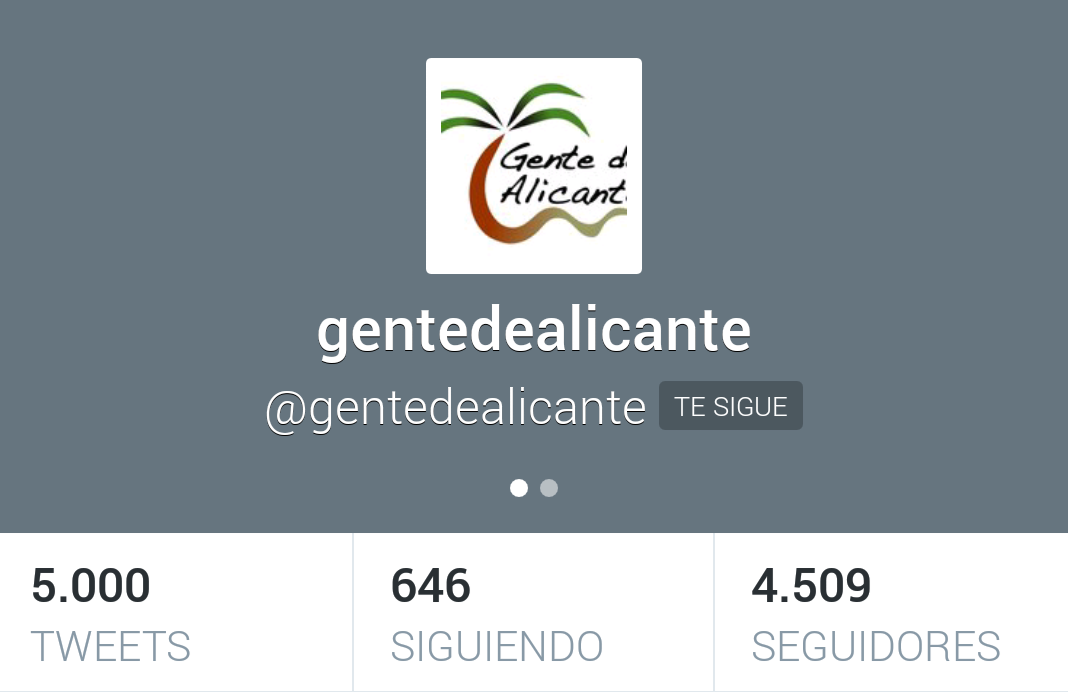The image depicts a screenshot likely from a mobile device, displaying a profile from a social media platform in a non-English language. The background is gray with a prominent white square at the top center, showcasing a logo that resembles a palm tree with green and brown squiggly lines. The text within the white square is partially cut off but reads "Gente d Alicante," stylized as "G-E-N-T-E D A-L-I-C-A-N-T-E."

Below the logo, in white lettering, the profile name "Gente de Alicante" is repeated along with the handle "@GenteDeAlicante." The profile statistics underneath include 5,000 tweets, 646 following ("seguiendo"), and 4,509 followers ("seguidores"). On the lower part of the gray portion, there are two small dots suggesting the presence of additional images or content that can be navigated to, typical of a carousel feature. Overall, the screenshot appears to be from a mobile website or app, focusing on the social media presence of "Gente de Alicante."